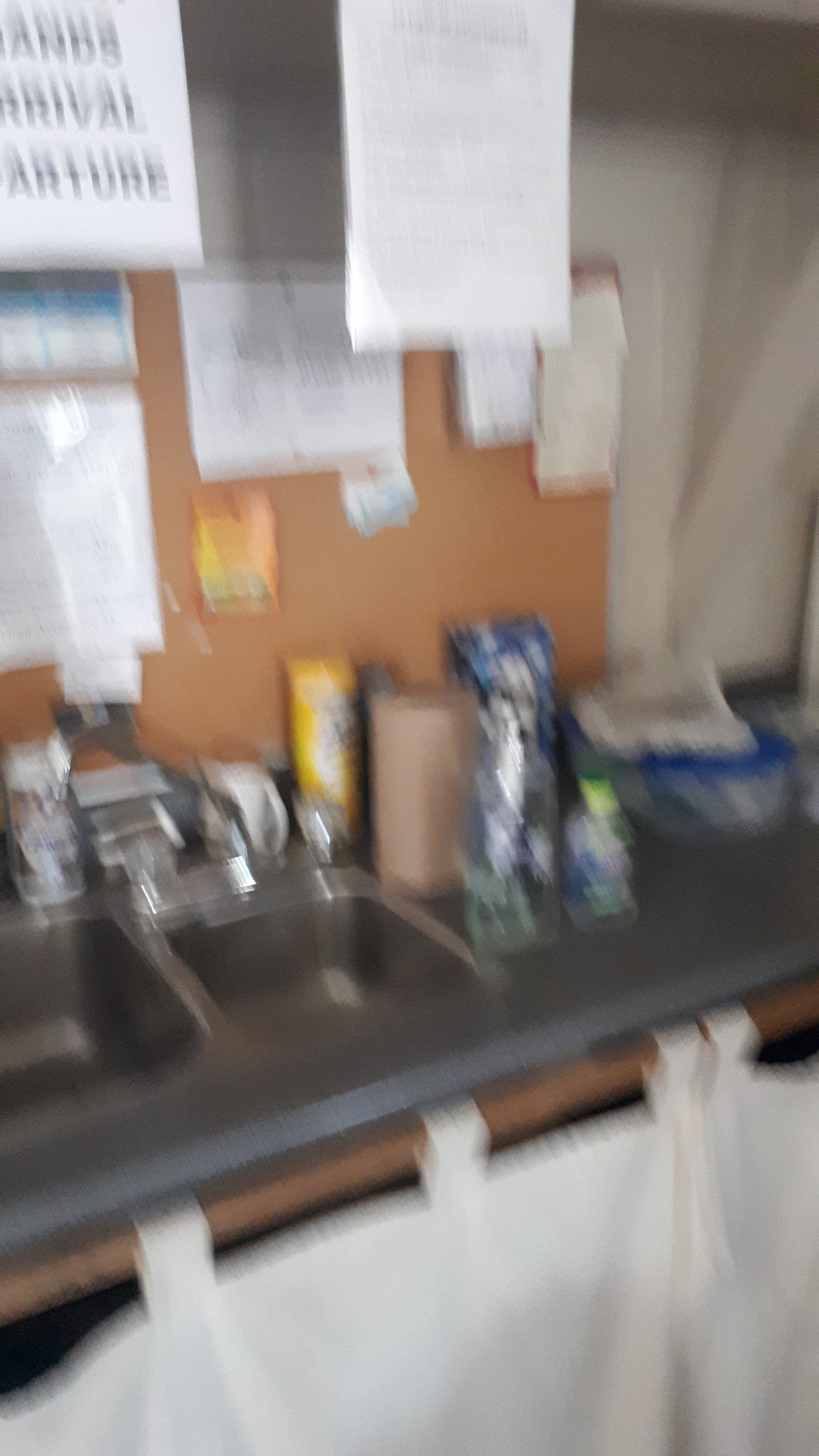This blurry photograph captures a cluttered scene featuring a gray countertop with two small silver sinks, possibly in a commercial setting like a restaurant. The sink area appears empty, but surrounding it are various jars and a short, yellow bottle, which might be a cleaning product or hand sanitizer. To the right of the sink, several items crowd the space, including what looks like a brown bag, paper towels, and a blue and green bag. Above the counter, there’s a tan-colored wall that darkens in the shadows, with a cork bulletin board pinned with multiple papers of varying shapes and sizes, some encased in plastic. Specific items on the board include a dark blue and light blue striped paper and another orange and yellow paper. Hanging above, there are two white signs with black, illegible lettering, and another piece of paper with blue ink reading partially legible words like "Arrival" and "Archer." Below the countertop, white curtains with fabric tabs hang from a wooden dowel, replacing cabinet doors. The overall image is marred by significant blurriness, making it difficult to decipher precise details, but the scene combines a mix of organizational chaos and utilitarian elements typical of a busy, functional workspace.